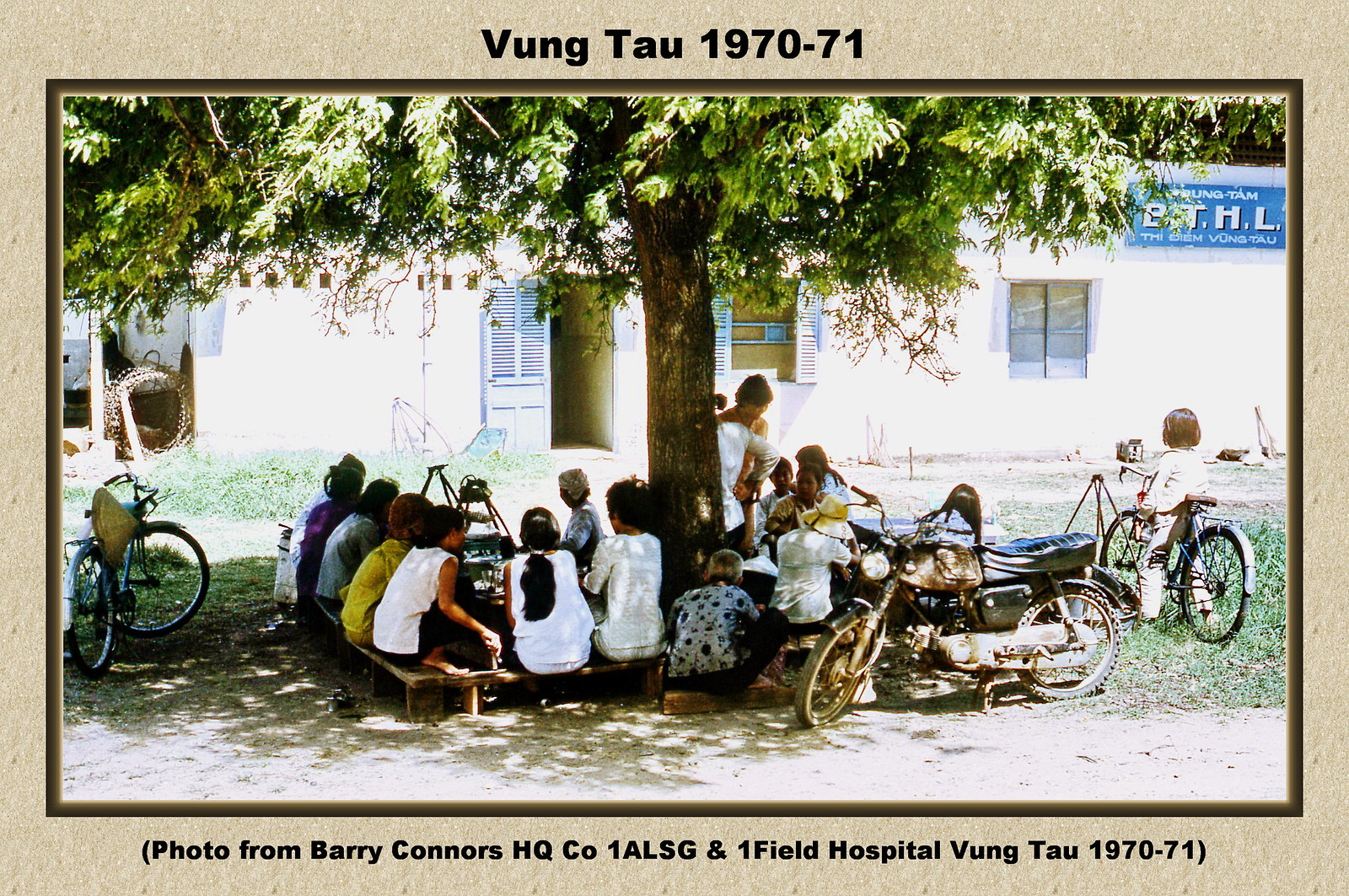A sunlit, outdoor scene from Vung Tau 1970-71, captured in a photograph framed by a tan border with a thin brown line. The top of the frame reads "Vung Tau 1970-71" and the bottom states, "Photo from Barry Connors HQ CO 1 ALSG and 1 Field Hospital Vung Tau 1970-71." The image portrays a group of women and children lounging on low benches under the dense, leafy canopy of a central tree, providing ample shade. They are facing inward, engaged in a communal moment. Surrounding them are several bicycles, including a prominent black and silver motorcycle in the foreground. Behind the group, a white building with blue shutters and trim, and an obscured sign that partially reads "B-T-H-L" is visible, adding a touch of architectural detail to the vibrant social setting.